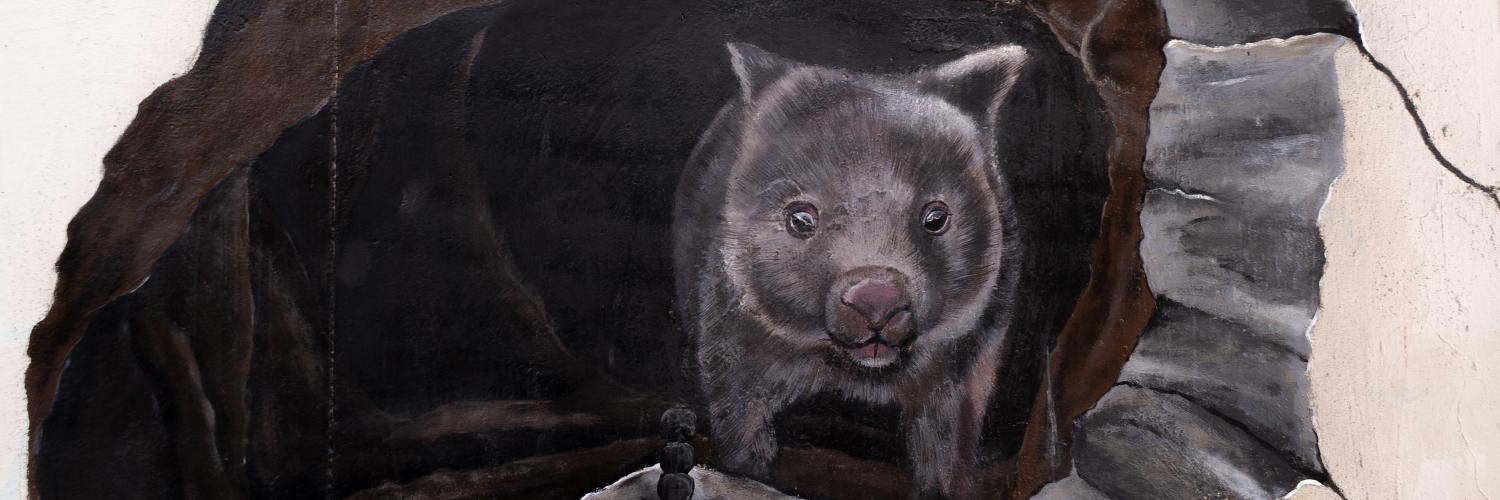The image depicts a painting of an ambiguous animal emerging from a cave, featuring an outdoor setting. The creature has a disproportionately large head, short stubby legs, pointy triangular ears, and small black eyes with a hint of pink around them. Its fur sports a grayish-brownish color palette. The setting includes the cave's brown interior and lighter colored stones visible on the right-hand side outside of the cave. The animal seems to be gazing directly out of the cave with a somewhat abstract or poorly-drawn appearance. The unclear identity of the animal, resembling elements of a bear, pig, wolf, or even a rabbit at first glance, adds an element of mystery to the painting.